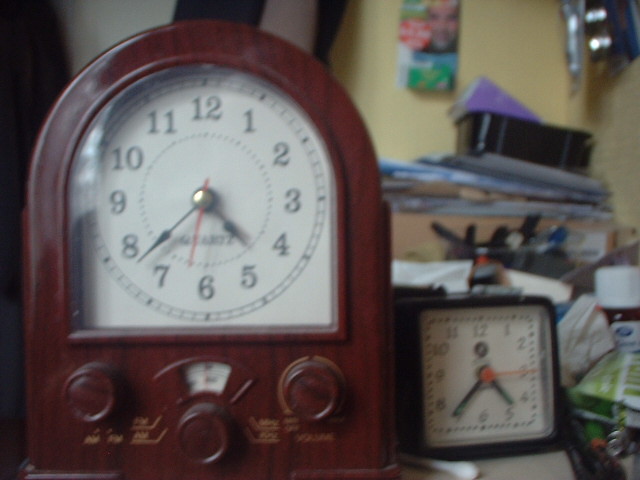This close-up photograph captures a cluttered table dominated by two distinctive clocks. On the left, there's an old-fashioned mantel clock-radio hybrid, encased in dark mahogany wood with an arched top and flat base. The face of the clock is white with black numbers and hands, alongside a smaller red second hand, all anchored by a brass pivot. Below the clock face, the radio section of the piece displays wooden dials, dark brown like the casing, with gold lettering indicating functions such as AM and FM tuners, volume controls, and other markings obscured by blur and shadow.

To the right of the mantel clock, a smaller, square-shaped alarm clock features a black housing with a contrasting white face. Its black hands show the hour close to 4:37, with a distinctive red second hand overlapping between the minute markers 6 and 7. Surrounding these clocks, the table is strewn with various objects, including stacks of white, dark blue, and light brown papers, a black crate, a cylindrical bottle with a white label, and a pill bottle with a white lid. The yellow wall behind the table holds a magazine showing a man's face against colorful elements and an additional silver object, adding to the overall sense of clutter.